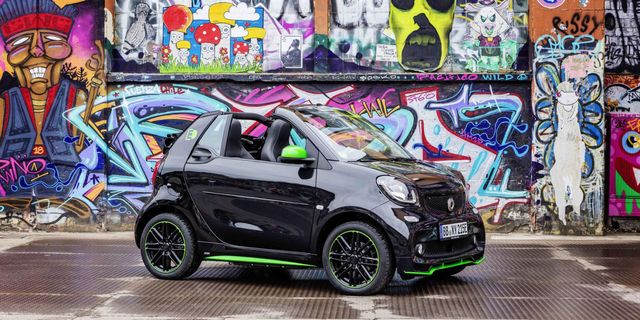This photograph features a tiny, glossy black, two-seater electric car with striking lime green accents on the bottom of the doors, the front grille, and the side mirrors. The car is parked on a surface that looks like concrete or possibly a metal grate. Behind it stands a vibrant wall adorned with a riot of colorful street art and graffiti. The art includes a vivid green skull that seems to be yelling, a striking portrait of a man with a red bandana and blue vest grinning broadly, and various bright mushrooms in hues of pink, blue, purple, and white. There’s also a ghostly white figure and other intricate graffiti designs. The car itself features a long, rectangular European-style front tag and a small, round hood emblem, although the make of the car remains unidentified. While the car's compact and cute design is eye-catching, its small size suggests potential vulnerability in collisions.